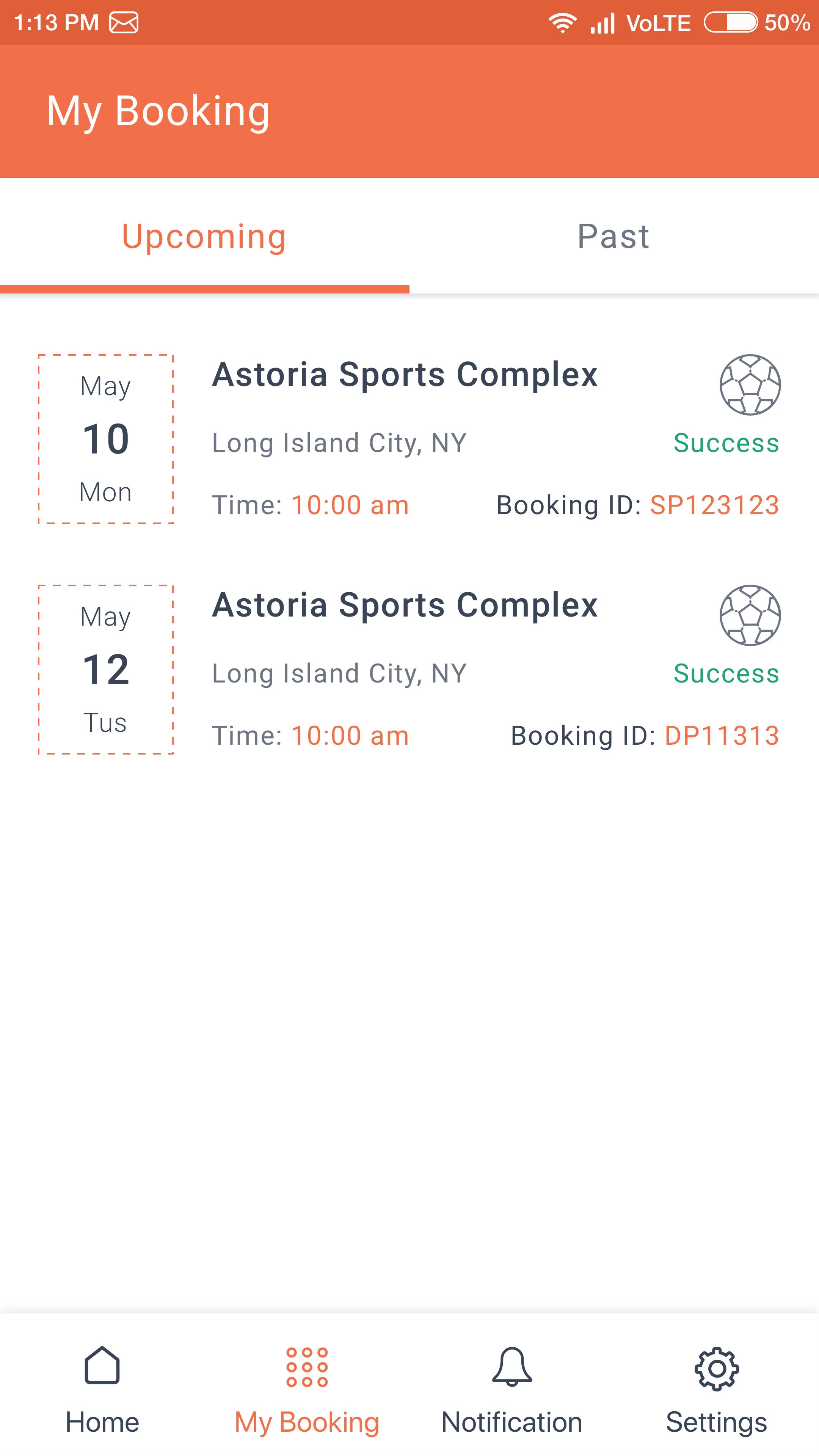The image captures a screenshot of a mobile booking app taken at 1:13 PM, with the battery level at 50%. The header of the app is highlighted in orange with the words "Upcoming" and "Past"; "Upcoming" is marked in orange and "Past" in gray. Listed are two bookings:

1. **May 10th, Monday (MON)**:
   - **Location:** Astoria Sports Complex, Long Island City, New York
   - **Contact Person:** Tom
   - **Time:** 10:00 AM
   - **Booking ID:** SP-123123 (displayed in red)
   - **Status:** Success (displayed beneath a soccer ball icon in green)
   
2. **May 12th, Tuesday (TUE)**:
   - **Location:** Astoria Sports Complex, Long Island City, New York
   - **Contact Person:** Tom
   - **Time:** 10:00 AM
   - **Booking ID:** DP-11313
   - **Status:** Success (displayed beneath a soccer ball icon in green)

At the bottom of the screenshot, there are navigation icons labeled as Home, Mob Booking (in red), Notification, and Settings.